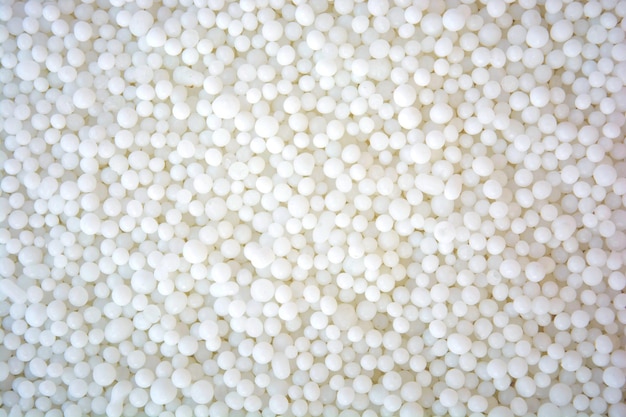The image showcases an extensive close-up of numerous small, shiny white spheres varying slightly in size, reminiscent of pebbles or beads. These spheres, potentially as small as BB pellets or akin to Dippin' Dots ice cream bites, densely fill the entire frame, leaving no empty space. Their slight translucency and solid white color give them a unique appearance that might be comparable to crafting styrofoam balls. Shadows are subtly present in the corners, especially in the top left and bottom right, adding depth to the image. The uniformity and sheer number of these quarter-to-nickel-sized spheres, consistently spread across the entire picture, present an intriguing and almost hypnotic pattern that draws the viewer in.